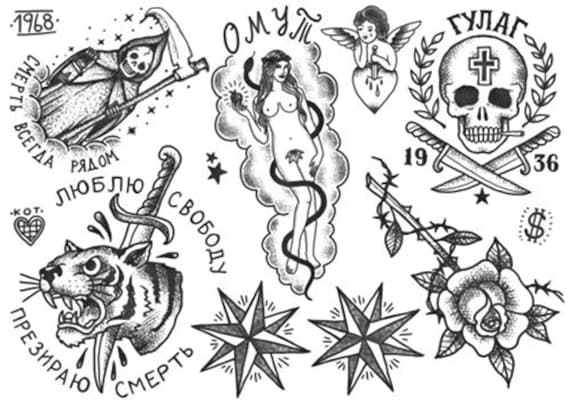This black-and-white digital montage features a series of ominous tattoo patterns accompanied by Russian text. At the top left, there's a depiction of the Grim Reaper wielding an axe. In the center, a snake coils around the body of a naked woman. Below her, two stars are positioned. The bottom left showcases a tiger's head, pierced by a sword with blood emerging from the wound. On the top right, an angel is illustrated piercing a heart with a sword. Next to it, a skull with a cross on its forehead is flanked by two leaves and accompanied by two crossed knives and the year "1936." The bottom right corner presents a rose with intertwining vines and visible thorns. Additionally, a dollar sign and other unreadable phrases in Russian are scattered throughout the image. The phrases "1968" and "Ami" are visible among the intricate designs.